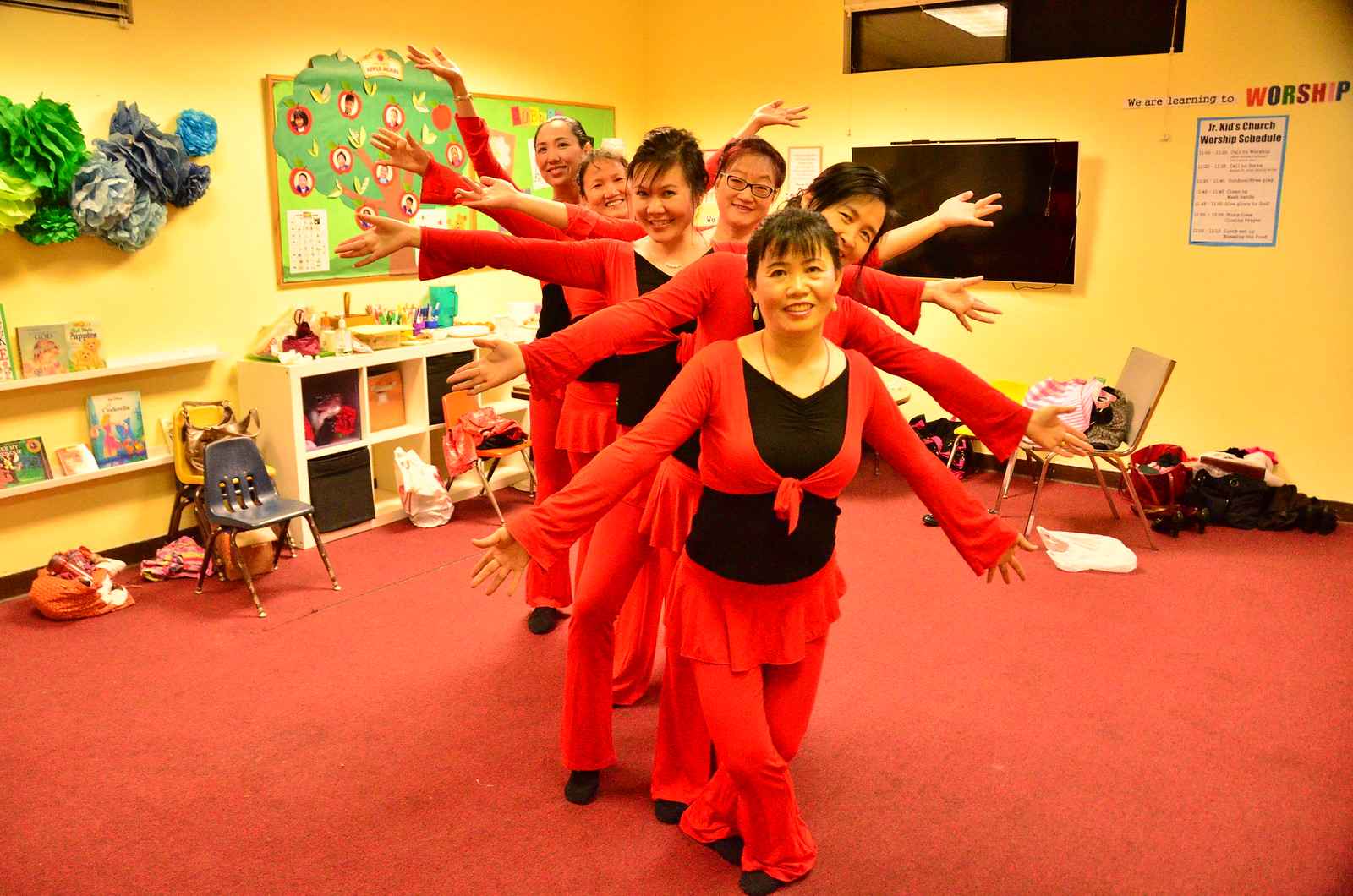The image is a color photograph in landscape orientation, depicting six Asian women in a classroom with yellow walls and a red carpeted floor. The women, who appear to be in their 20s to 40s, are aligned in a row from front to back, all wearing matching outfits consisting of red long-sleeved tops, black t-shirts underneath, red trousers, red skirts over the trousers, and black footwear. They are looking at the camera with outstretched arms, creating a visually flowing effect as each woman's arms are progressively raised higher from front to back. The classroom setting includes a green poster board with photos on the left side, white shelves underneath, and various items around the room. On the right side of the wall, there is a black t-shirt mark, and additional details like a tissue paper display and a tree picture with photos of children inside red apples can be seen in the background, further emphasizing the educational environment.